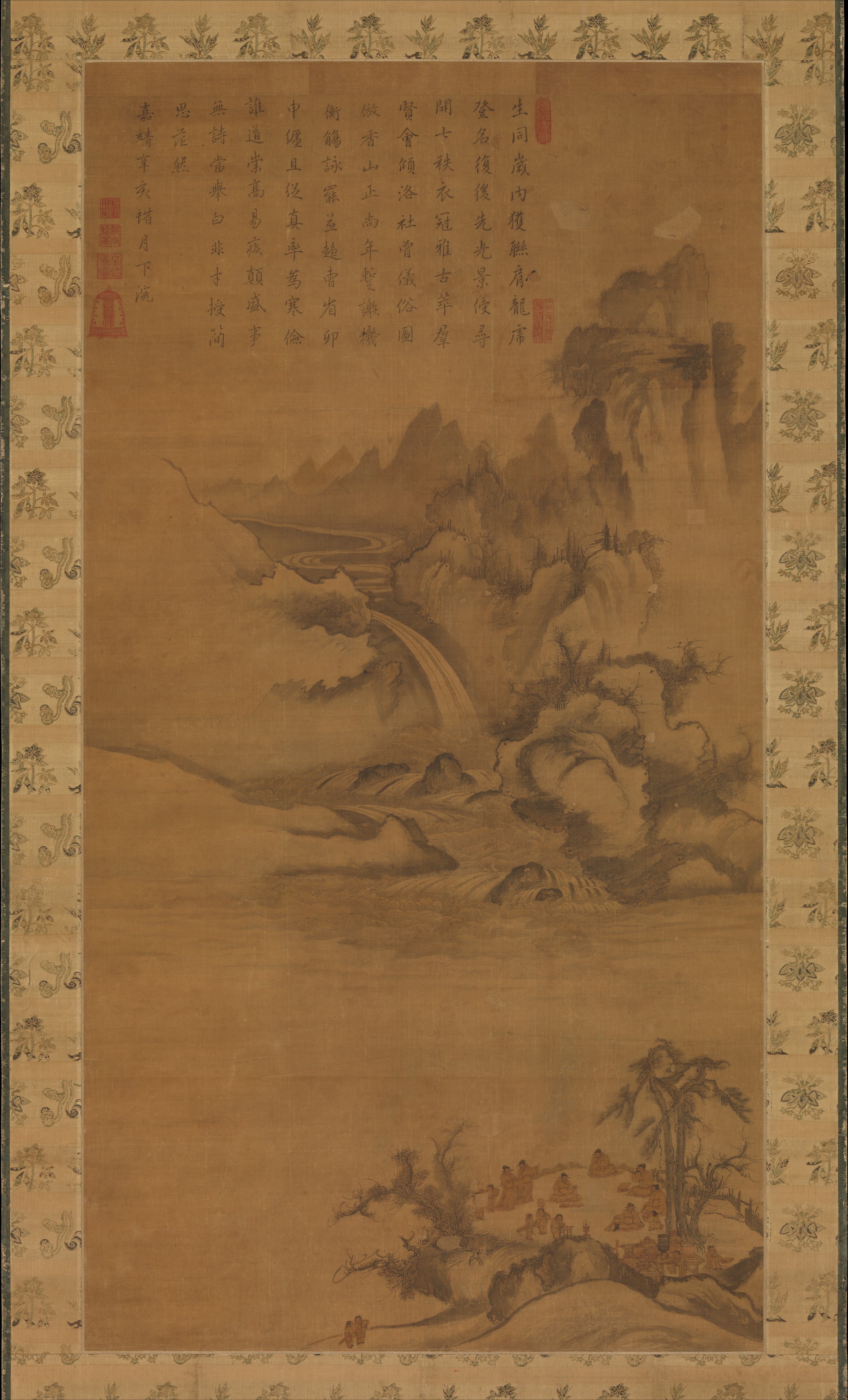This image captures a highly detailed photograph of an old, vertical Asian scroll, possibly serving as a decorative poster or even a calendar. The piece appears to be crafted on a parchment or scroll-like material with a beige foundation. Surrounding it is a border adorned with intricate, black sketches of plants, flora, and perhaps additional figures that encompass the artwork.

The centerpiece of the scroll begins in the upper left corner, featuring rows of Korean or Chinese characters inscribed in black ink. Directly below the text, the central expanse of the artwork presents a meticulously hand-drawn landscape. This scenic portrayal includes mountainous terrains on the right side, transitioning into a valley with a river that cascades into a waterfall, before continuing forward as a wavy stream. 

Situated in the bottom right portion of the artwork, another landscape scene unfolds. Here, a serene depiction includes a couple of trees and several figures gathered in a clearing. Some of these figures can also be seen down to the left of this area, potentially monks or individuals in robes, engaged in some communal activity within a tranquil, verdant setting. The artwork's palette largely comprises shades of gray, light and dark browns, red, and black, contributing to its rich, artistic presentation. The overall impression is a vertical rectangular scroll featuring a harmonious blend of nature, human elements, and traditional Asian script.